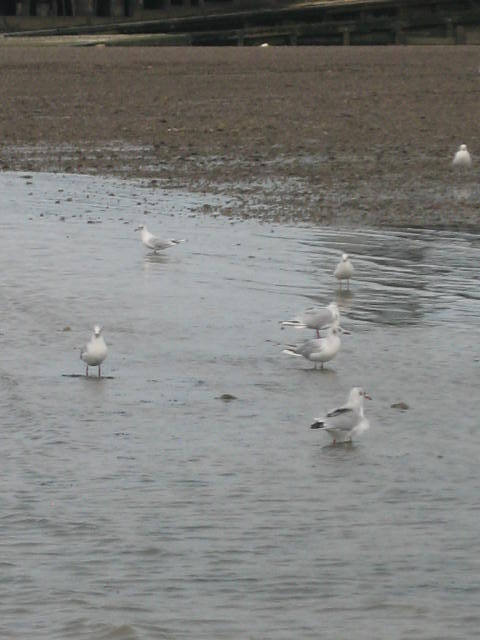This outdoor photograph captures a scene in a shallow body of gray, muddy water at what appears to be the edge of a small pond or river near a beach. The photographer, likely standing in the water, frames seven small white and gray birds, possibly seagulls or ducks, with six standing in the water and one on the shore. The shoreline, covered with small brown rocks or dark sand, stretches into the distance. Prominent in the background is a large bridge or overpass made of concrete or stone, extending from the left to the right side of the image, suggesting proximity to an interstate. The overall ambiance is dull, with the water and surroundings lacking vibrant colors.